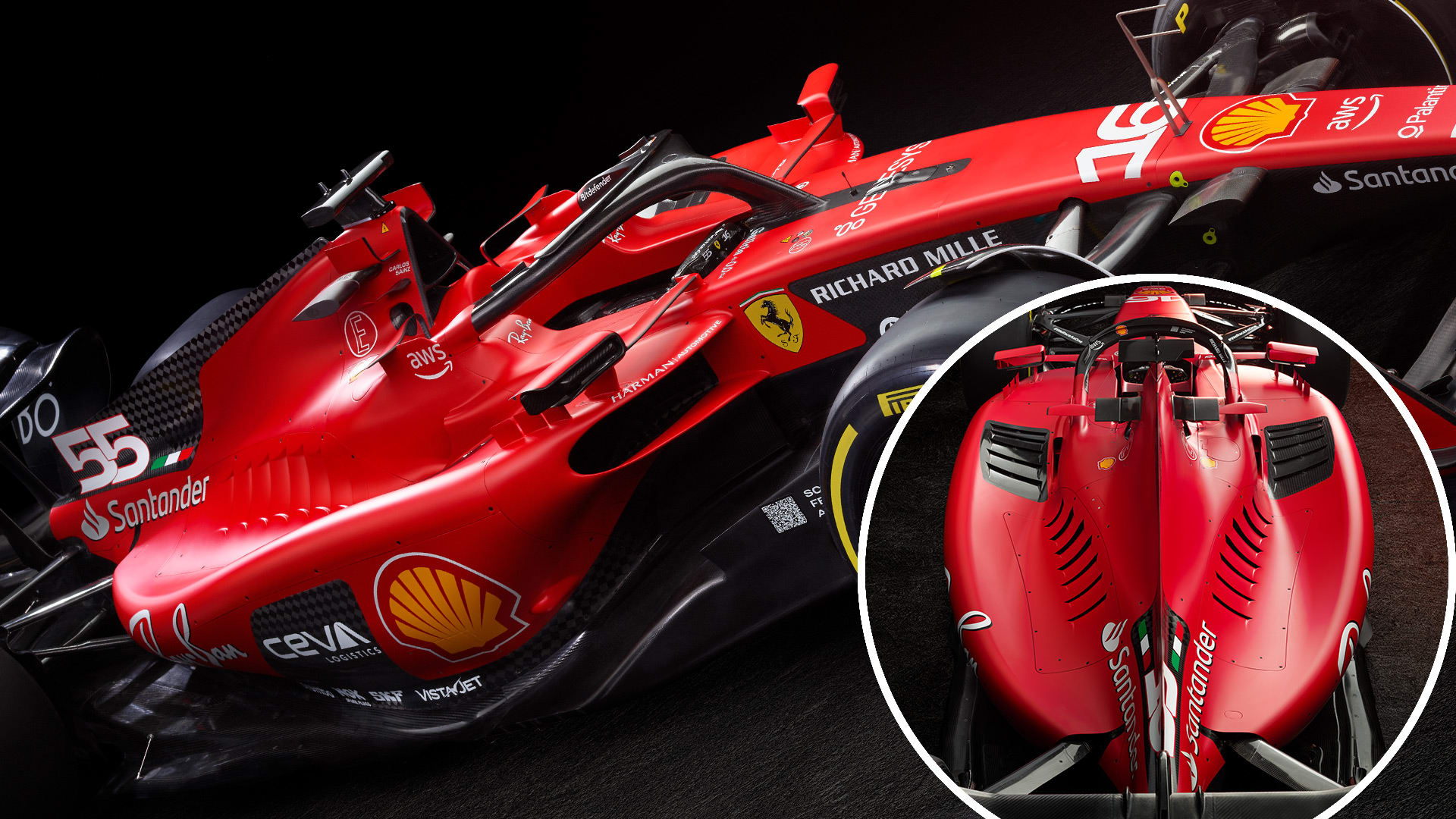This image showcases a bright red, fire-engine colored Ferrari Formula One racing car. The car is adorned with several sponsor logos, including prominent ones like Shell, Santander, CEVA, and Ray-Ban. The name "Richard Mille" (incorrectly spelled as "Mill" in one description) is visible on the side, highlighting the luxury watch sponsor rather than the driver's name. The car sports the number 55, which is displayed prominently on various angles, including a front-on-side view and a smaller top-down image in the corner. The car's low-slung, aerodynamic design is accentuated by black accents and is clearly engineered for high-speed racing. Other notable details include a barcode and intricately placed sponsor logos endorsing brands like Amazon alongside CEVA Logistics. The vehicle’s sleek design and vibrant color scheme make it unmistakable on the racetrack.